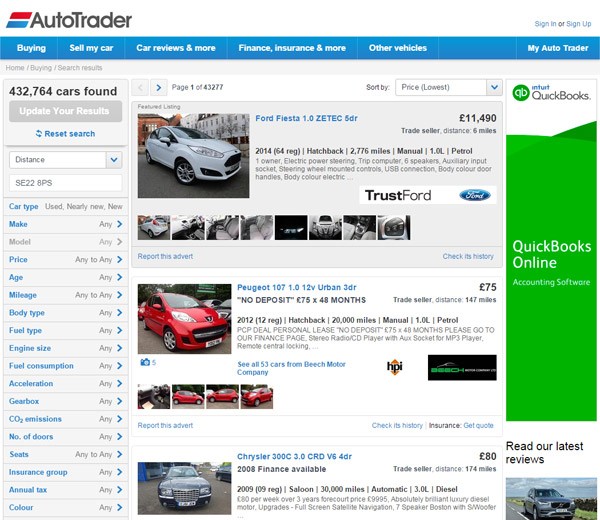The screen capture presents the homepage of AutoTrader, displaying the website's various tabs at the top which include: Buying, Sell My Car, Car Reviews & More, Finance, Insurance & More, Other Vehicles, and My AutoTrader. The search results indicate a total of 432,764 cars found. On the first page, the listings begin with a white 2014 Ford Fiesta, followed by a red 2012 Peugeot 107, and a 2008 Chrysler 300C. To the left of the car listings, a comprehensive filter section is visible, allowing users to specify their search criteria by make, model, price, age, mileage, body type, fuel type, engine size, fuel consumption, acceleration, gearbox, CO2 emissions, number of doors, seats, insurance group, annual tax, and color.